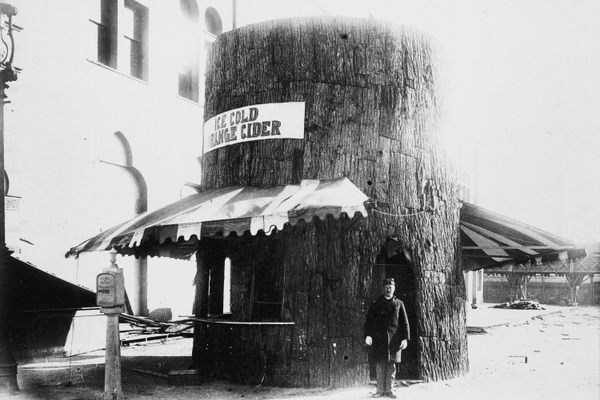This black-and-white photograph captures a uniquely crafted business establishment, featuring a cylindrical structure with a rough, tree-like texture. The structure, which appears to be either fashioned from or carved out of a massive redwood tree, serves as an "Ice Cold Orange Cider" stand. At its entrance stands a white man dressed in a black coat and matching hat, his arms resting calmly at his sides as he gazes directly at the camera. The door of the stand is distinctively shaped with an oval top rather than the typical rectangular form, adding to the whimsical charm of the scene.

Adjacent to this doorway is a window section with a counter, shaded by an overhanging canopy. Above the window, a white banner boldly announces "Ice Cold Orange Cider." The cylindrical structure extends a second canopy that nearly encircles the entire stand, lending additional shaded areas for customers.

In the left foreground, a parking meter is visible, adding a touch of urban context to the otherwise rural-feeling scene. Behind the stand, on the left side of the photograph, there's a building that fades into the background due to the bright white tones, giving the image an ethereal, dream-like quality. The combined elements create a captivating depiction of a quaint yet surreal commercial setup, offering a glimpse into a simpler time.